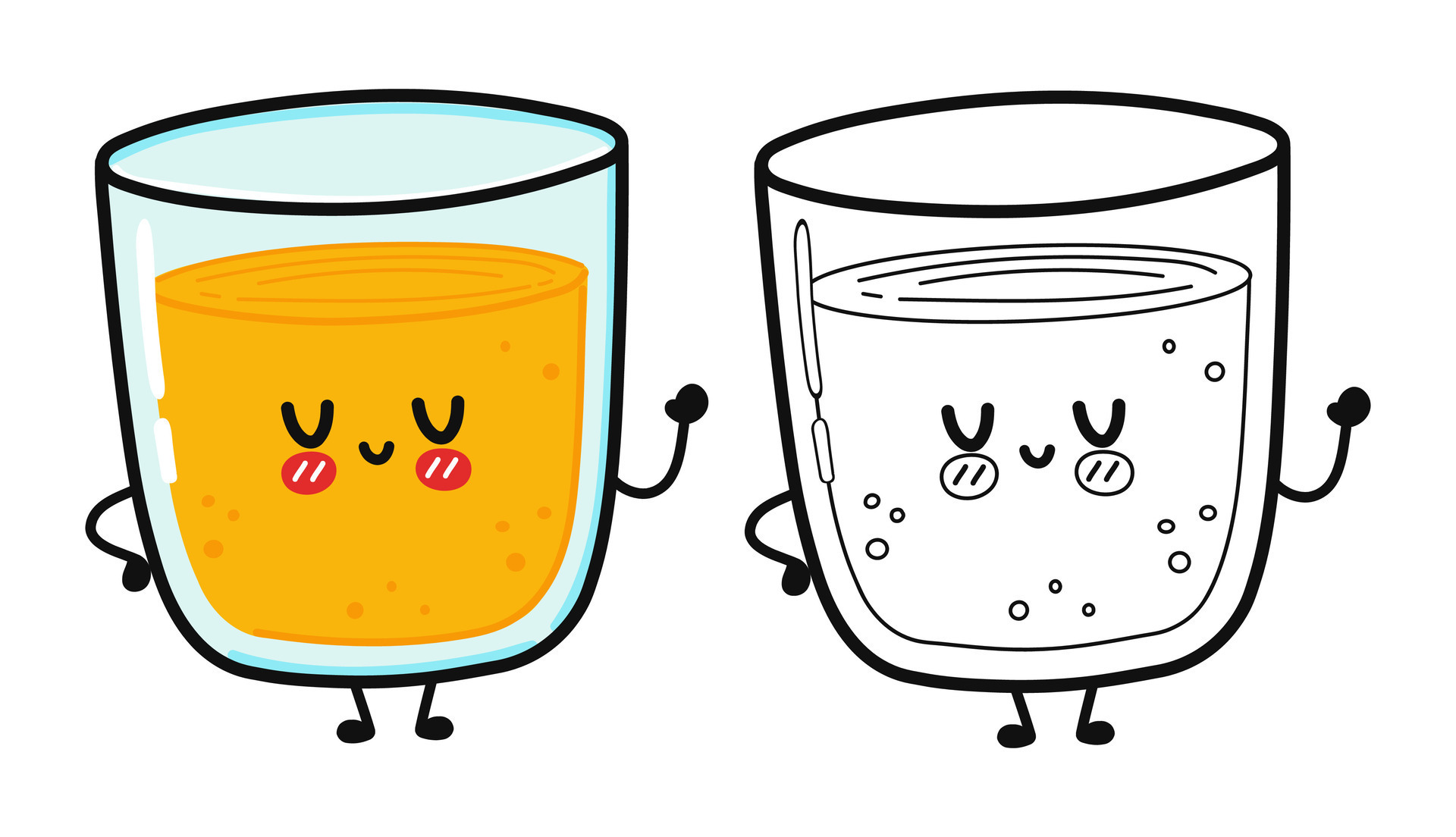The illustration depicts two cartoonish, anthropomorphized cups standing side-by-side on a white background. The cup on the left is a light blue, transparent glass with dark blue edges and black outlines. It is filled with a yellow liquid that has darker yellow bubbles and lines at the top. The cup features closed, black eyes, a black smile, and red cheeks with white stripes. The left hand is positioned on its hip, while the right hand is raised. It stands on black legs and feet.

The cup on the right mirrors the one on the left in terms of shape and features but is entirely in black-and-white line art. It contains a white bubbly liquid and also has black eyes, a smile, and simple stick-figure arms and legs. Both cups sport cheerful expressions and seem to be happily animated, as if enjoying a lively conversation.